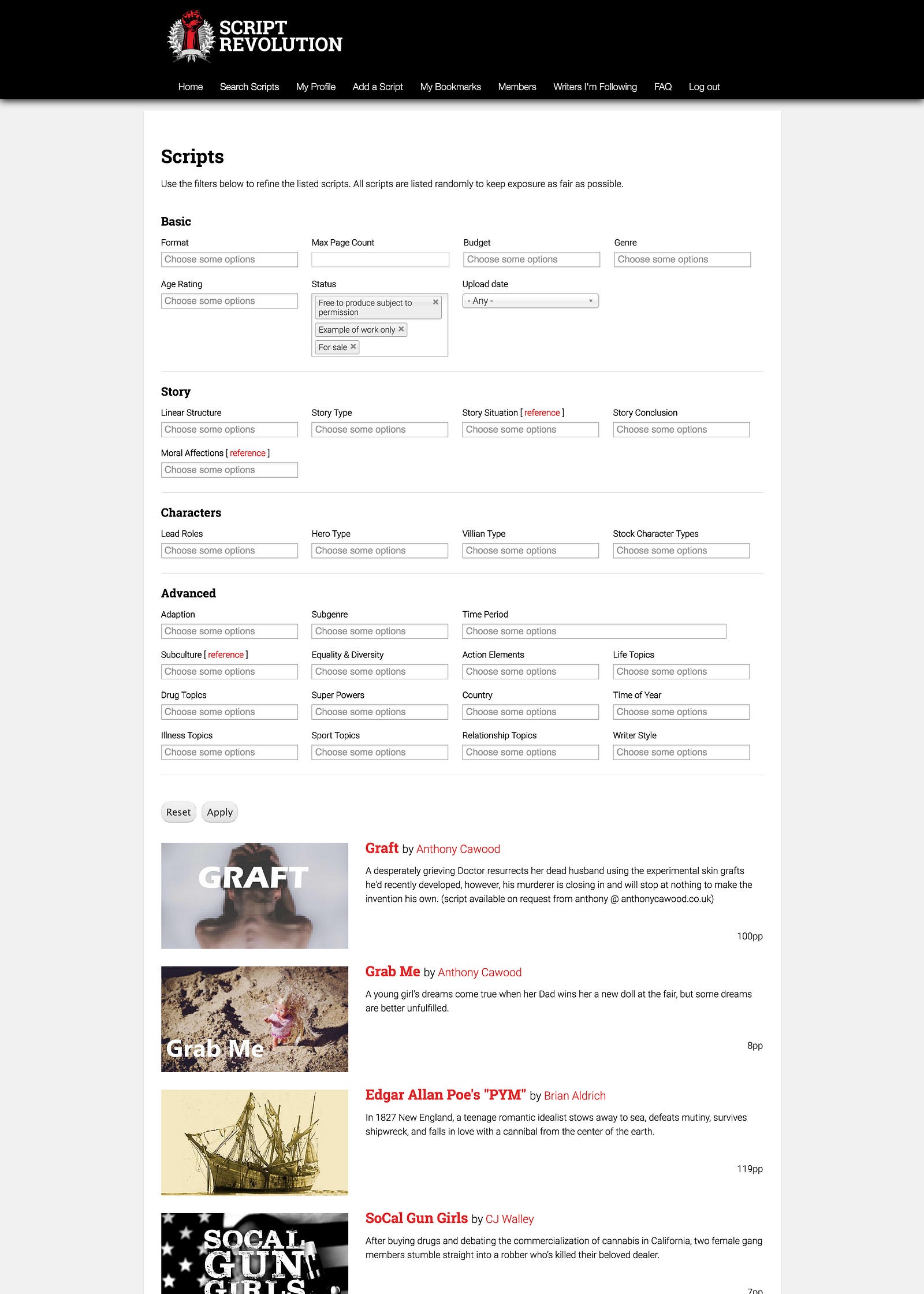The image is a vertical layout featuring the Script Revolution website interface. At the top of the image is a prominent black bar, adorned with the bold, white text "SCRIPT REVOLUTION" in all capital letters. Adjacent to the text is a striking icon: a red fist raised upwards, symbolizing strength or revolution, nestled between two white laurel leaves.

Immediately below this header, there is a navigation menu with various options arranged horizontally from left to right. These options are: "Home," "Search Scripts," "My Profile," "Add a Script," "My Bookmarks," "Members," "Writers I'm Following," "FAQ," and "Logout."

Underneath the menu, there is a large white box prominently titled "Scripts." This section advises users to utilize the filters below to refine the listed scripts, which are displayed randomly to ensure fair exposure. The box includes several fields for specific filtering options:

- **Basic Filters:**
  - **Format:** Options to choose from various script formats
  - **Max Page Count:** An empty field for the maximum number of pages
  - **Budget:** Different budget categories
  - **Genre:** Various genres to select from
  - **Age Rating:** Diverse age ratings
  - **Free to Produce:** Options for permission levels (e.g., "Subject to Permission," "Example of Work Only," "For Sale")
  - **Upload Date:** A range of dates

- **Story Filters:**
  - **Linear Structure:** Various structural options
  - **Story Type:** Different types of stories
  - **Story Situation:** Specific situational categories
  - **Story Conclusion:** Types of conclusions
  - **Moral Affections:** Moral themes or elements

- **Character Filters:**
  - **Lead Roles:** Various lead role types
  - **Hero Type:** Different hero archetypes
  - **Villain Types:** Different villain archetypes
  - **Character Types:** Specific character traits or roles

- **Advanced Filters:**
  - **Adaptation:** Options for adaptations
  - **Subgenre:** Various subgenres
  - **Time Period:** Different historical periods
  - **Subculture:** Diverse cultural contexts
  - **Equality and Diversity:** Themes of equality and diversity
  - **Action Elements:** Various action elements
  - **Life Topics:** Topics that deal with aspects of life
  - **Drug Topics:** Elements involving drugs
  - **Superpowers:** Options involving superpowers
  - **Country:** Specific countries
  - **Time of Year:** Different seasons or times of the year
  - **Illness Topics:** Topics involving illness
  - **Sport Topics:** Elements related to sports
  - **Relationship Topics:** Topics about relationships
  - **Writer's Style:** Various writing styles

This detailed layout facilitates users in thoroughly searching and filtering the scripts available on the Script Revolution platform.